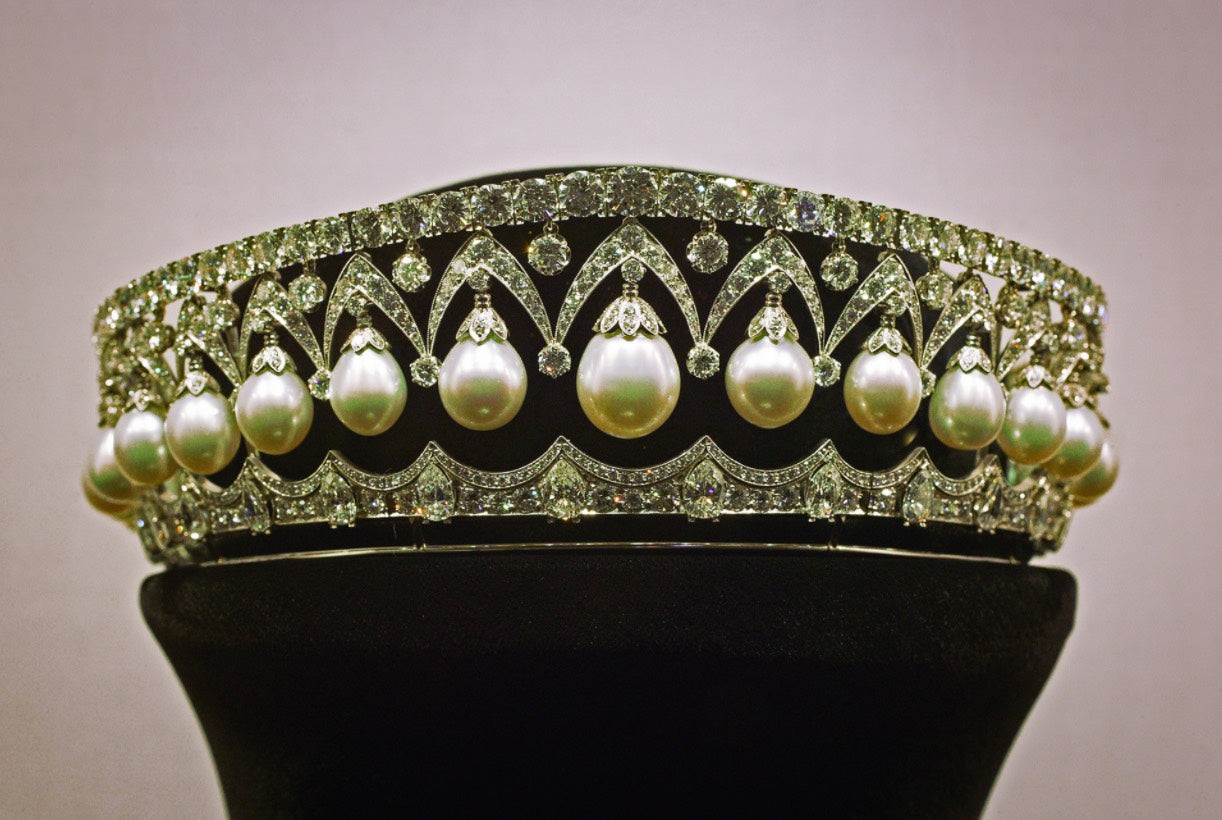This image captures a close-up of an exquisite crown displayed on a black velvet pedestal against a plain white background. The crown, likely to be a piece of royal jewelry, is approximately six inches tall and features a circular, flat design with intricate detailing. Adorned with a plethora of large pearls, each spaced about two inches apart, these pearls dangle delicately from gold flower-like settings. These gold elements connect to the outer ring of the crown through M-shaped gold structures. Additionally, the crown is adorned with a multitude of diamonds and possibly other precious jewels, including colored gems at the base, set within the intricate gold framework. The overall craftsmanship of the crown, embellished with pearls, diamonds, and gold, speaks to its elegance and likely signifies it as a regal piece intended for a woman.